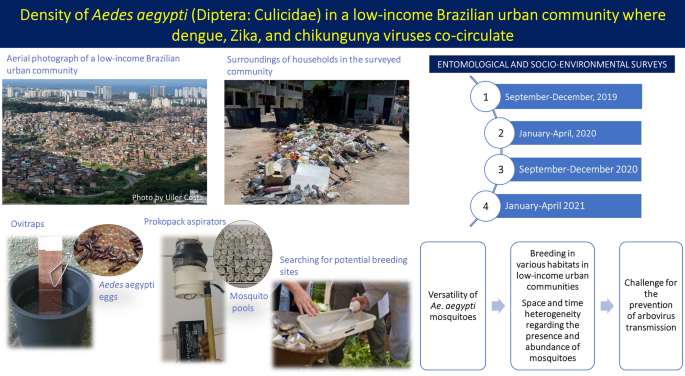The infographic details the density of *Aedes aegypti* (Diptera: Culicidae) in a low-income Brazilian urban community where Dengue, Zika, and Chikungunya viruses co-circulate. The background of the infographic is white, with a blue bar at the top featuring the title in yellow text. The top image is an aerial photograph labeled "Aerial photography of a low-income Brazilian urban community," showcasing a cityscape with gray buildings, brown residential houses, and green vegetation. Below, an image labeled "Surroundings of households in the suburban community" depicts a street strewn with trash, including white bags, brown paper, yellow items, and cardboard boxes, set against a backdrop of houses. 

Further down, the infographic shows various equipment used for entomological studies, including UV traps and Prokopack aspirators, and illustrates the life cycle of mosquitoes with images of larvae and breeding sites like buckets of water. Two workers can be seen using syringes to collect water samples, searching for potential mosquito breeding sites. The infographic also outlines "Entomological and socio-environmental surveys" conducted from September 2019 to April 2021, divided into four periods: September-December 2019, January-April 2020, September-December 2020, and January-April 2021.